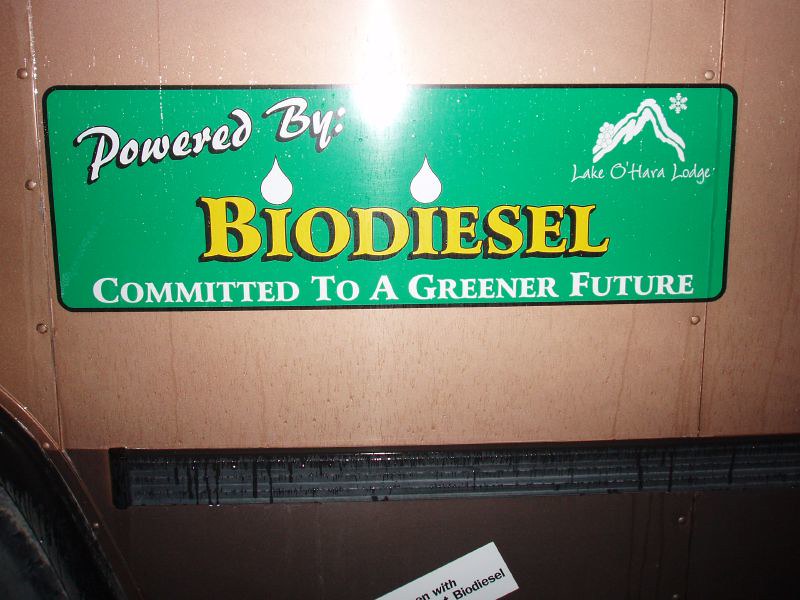In this zoomed-in image, we see the side of a truck or vehicle, with a focus on a green sign positioned centrally. The green sign, with rounded edges and a thin black border, reads "Powered by Biodiesel, Committed to a Greener Future" in various fonts. The lettering on the sign includes "powered by" in white text with black shadowing, "biodiesel" in yellow font with black shadowing, and "committed to a greener future" in white font. This sign is set against a beige wooden paneling or metal surface that appears brown or golden with rivets, and possibly damp with visible water drips. The upper right corner of the image also features a logo of a mountain labeled "Lake O'Hara Lodge." At the bottom, a partially visible, cut-off sticker hints at another biodiesel-related message. The bottom left corner shows a wheel, while a black rubber stripe runs horizontally with water droplets hanging from it. The colors in the image include shades of brown, light brown, black, white, green, and yellow, giving it an outdoor and somewhat industrial feel.